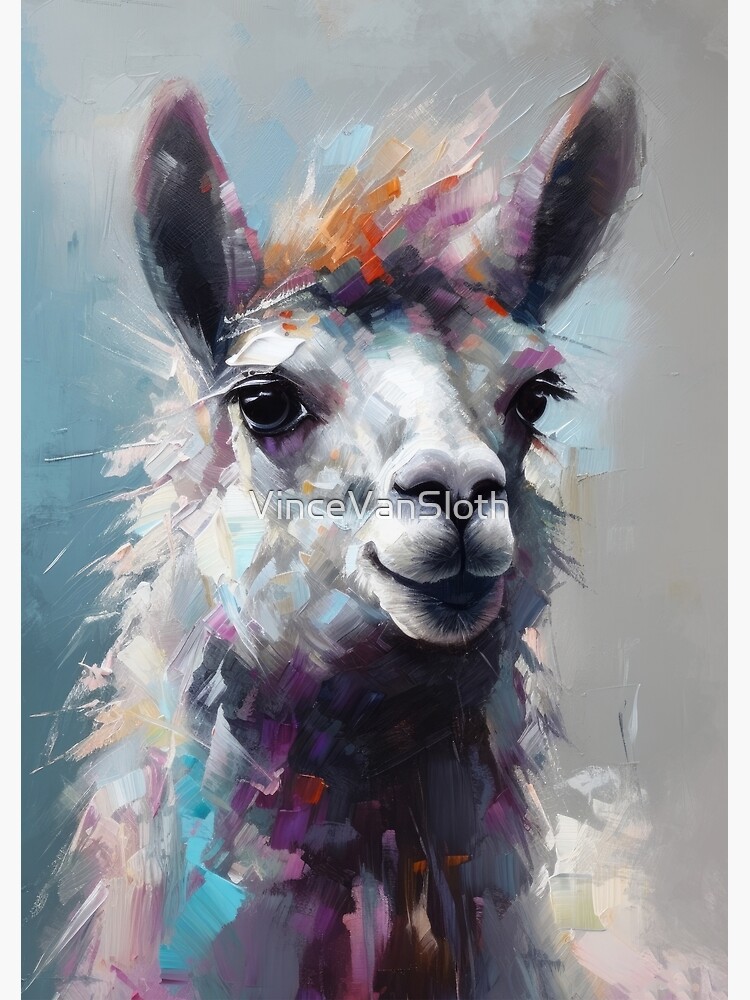This vertically aligned rectangular digital painting, resembling a poster with thin white borders on either side, features a close-up of a colorful llama against a blended bluish-gray background. The llama's face is predominantly white, with large expressive black eyes. Its ears are a mix of black, purple, and gray, while the hair between the ears bursts with vibrant splashes of orange, red, and purple. The chest and neck area of the llama showcase a dynamic mix of black, dark purples, reds, lighter purples, and some blues, contributing to the striking splash artwork style. Overlaying the center of this vibrant image in white text is the name "Vince Van Sloth."